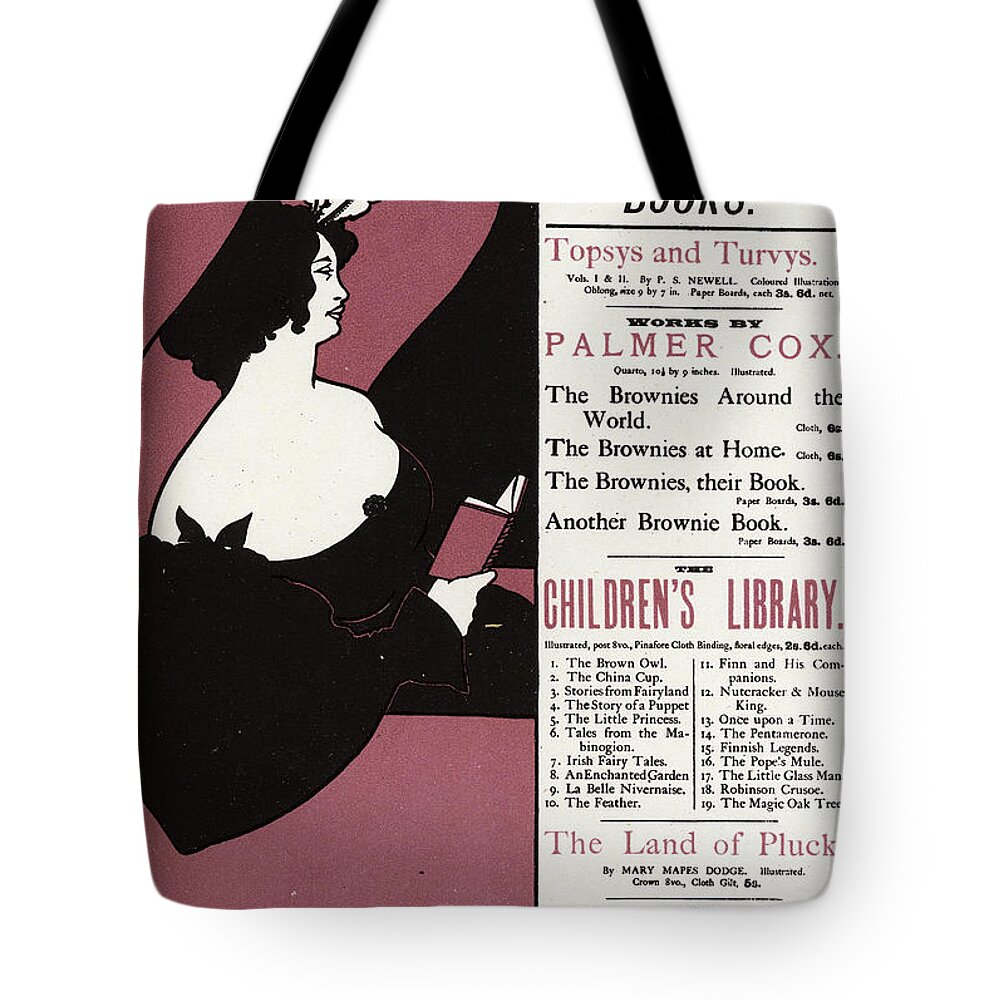This image features a stylish rectangular tote bag with a black strap handle and a rich burgundy background. The left side of the tote bag showcases a stylized black-and-white cartoon drawing of an elegant woman from a vintage era, possibly the 1950s. She has short, curly black hair and is wearing an off-the-shoulder black dress with poofy sleeves. She is depicted holding an open book that matches the burgundy background, adding a touch of sophistication to her look. The right side of the tote bag is densely covered with text in black and burgundy fonts, resembling a vintage newspaper printout. The text prominently features the titles "Topsy's and Turvy's" and "Works by Palmer Cox," listing various classic children's book titles such as "The Brownies Around the World," "The Brownies at Home," "The Brownies, Their Book," and "Another Brownie Book." Additional descriptions suggest the item belongs to a 'Children's Library' collection, including further book titles like "The Little Princess," "Nutcracker and Mouse King," "Robinson Crusoe," among others. The detailed text emphasizes the literary charm and nostalgic appeal, making this tote bag both a fashionable and culturally rich accessory.